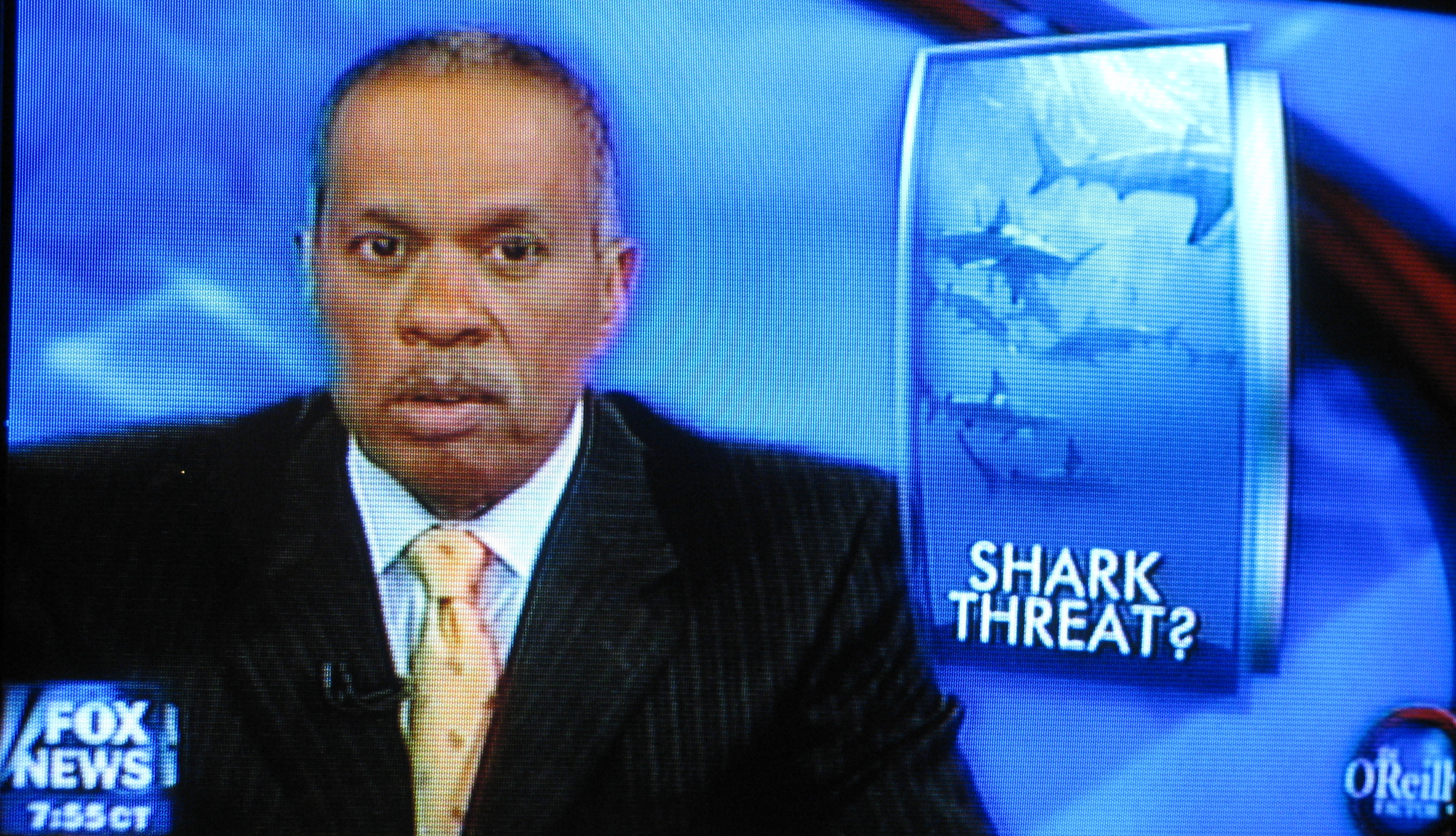The image is a landscape-oriented, color photograph of a television screen displaying a news program from Fox News Network. In the bottom left corner, the blue rectangle bears the white text "Fox News 755 CT," and in the bottom right, a blue circular logo reads "The O'Reilly Factor" in white text. The focal point is an African-American newscaster, likely in his late 50s or early 60s, positioned on the left side of the screen. He has salt-and-pepper hair, a gray mustache, and is looking slightly downward toward the viewer. He is dressed in a black pinstriped business coat, a light blue button-up shirt, and a distinctive yellow tie with dark yellow spots. Behind him, the background is predominantly blue. To his right is a superimposed rectangle featuring images of sharks with the bold, white text "SHARK THREAT?" The photograph appears to be a freeze-frame from the news segment, capturing the newscaster mid-broadcast.